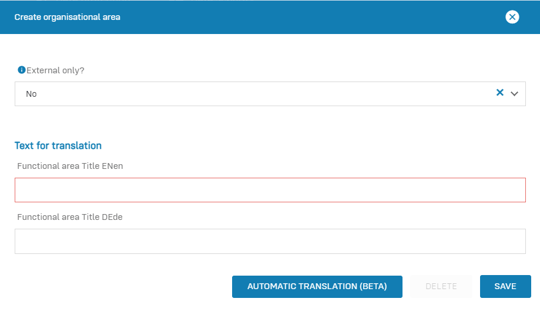In the image described, the background transitions from blue at the top, moving left to right, to white as it goes downward. Positioned at the top-left, in small white text on the blue background, are the words "Create, Organizational Area." A blank blue space follows this text. On the right side of this blue section is a white circle containing a blue 'X'.

Below this blue section, the background shifts to white. Towards the left side, there is a prominent blue circle featuring a white 'i' icon. Adjacent to this circle, in gray text, are the words "External Only?" Aligned beneath this is a drop-down box that spans horizontally across the section. Within this drop-down, the word "Noah" is written in black on the left, and a blue 'X' with a drop-down indicator is on the right.

Directly underneath, in blue text, it states "Text for Translation." Beneath this, in gray, it reads "Functional Area Title: ENen" — indicating English. A text field beneath this line is empty, meant for user input.

Further down, in black text, it says "Functional Area Title: DEde" — likely referring to German. There is another empty text box under this label for user input.

Towards the bottom-right of the image, there are two blue buttons. The first button reads "Automatic Translation (beta)." Adjacent to it, there is barely visible text that says "Delete." To the right of this, another blue button reads "Save and Wait."